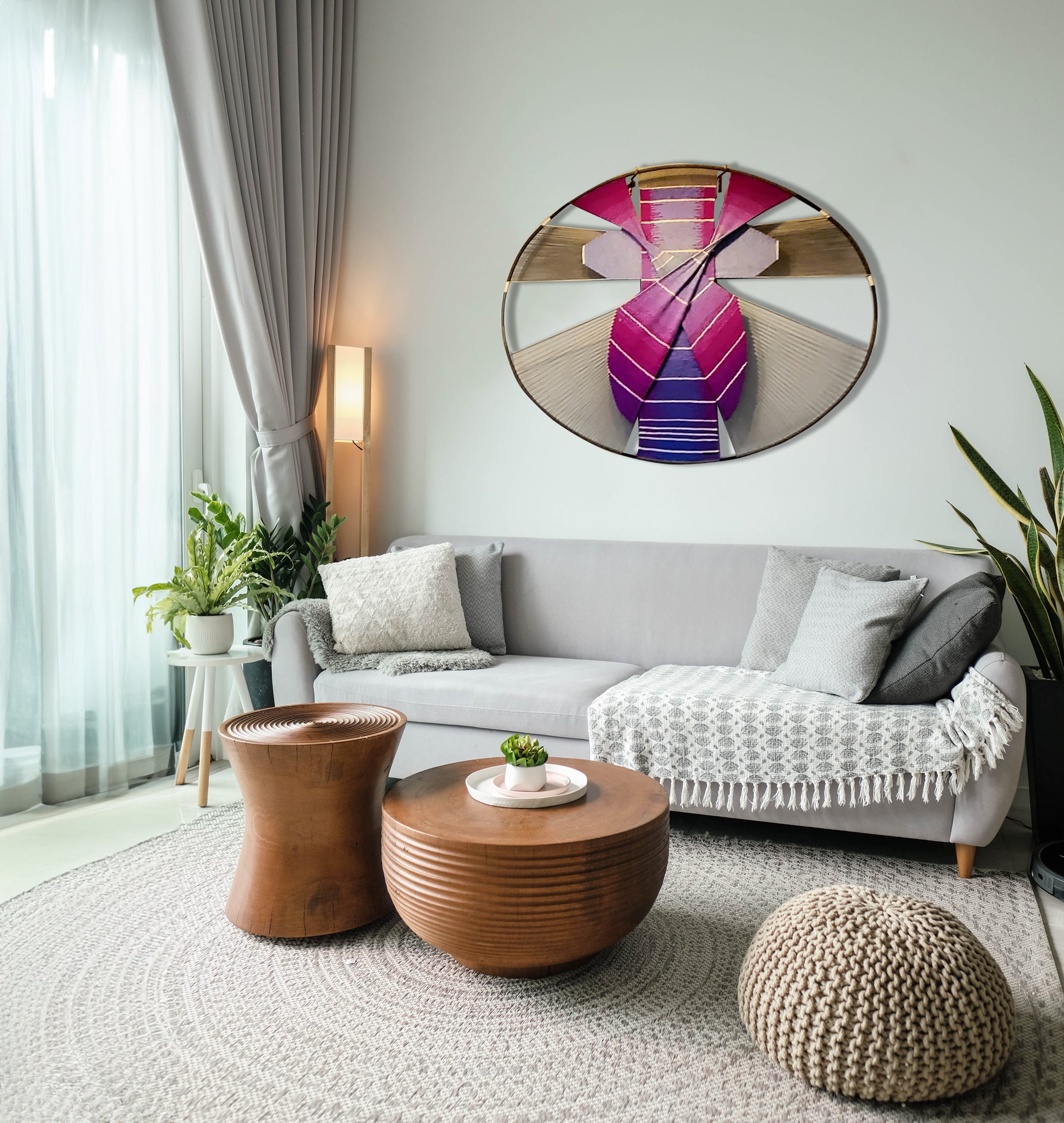The photograph depicts a well-lit, stylish living room bathed in natural light from a floor-to-ceiling window on the left, which is covered with sheer drapes and light beige curtains held back at the sides. Central to the room is a large off-white couch adorned with two gray and pale gray blankets, along with five throw pillows in shades of dark slate, pink, off-white, and gray. Above the couch hangs a striking piece of abstract art in an oval frame, featuring hues of pink, purple, blue, and brown. In front of the couch, two small, modern coffee tables—one round and one rectangular—sit on a large area rug that has a white and light blue circular pattern. Additionally, there is a crocheted off-white footstool and a small brown ottoman resembling a beanbag. Beside the couch, plants and a floor lamp add greenery and illumination to the space. To the right of the couch is another plant, creating a balanced and cozy ambiance in the room. The overall aesthetic is modern and inviting, characterized by a harmonious blend of neutral tones and vibrant artwork.